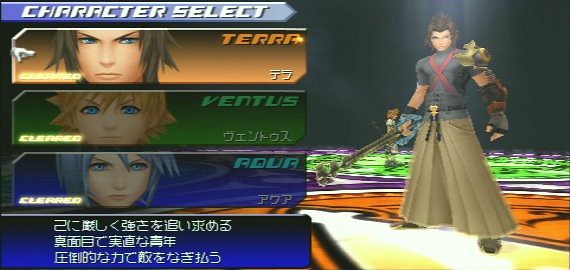This is a detailed screenshot from a Kingdom Hearts game, presented in a rectangular format that is wider than it is tall. On the left side of the image, a "Character Select" menu is visible, listing three characters: Terra, Ventus, and Aqua. Each character name is displayed in both English and stylized block letters, with Katakana text beneath them. All three characters are marked as "cleared." Below this list, there's a block of Japanese text written in white, superimposed on a gradient background that transitions from black to bright blue.

The right half of the frame features Terra, who is depicted standing with a Keyblade in hand. Terra is characterized by his muscular build and slightly spiky brown hair. He is dressed in wide pants and a shirt adorned with a prominent red "X" across the chest. The surface beneath Terra's feet is vividly colorful, adding a vibrant contrast to the scene.